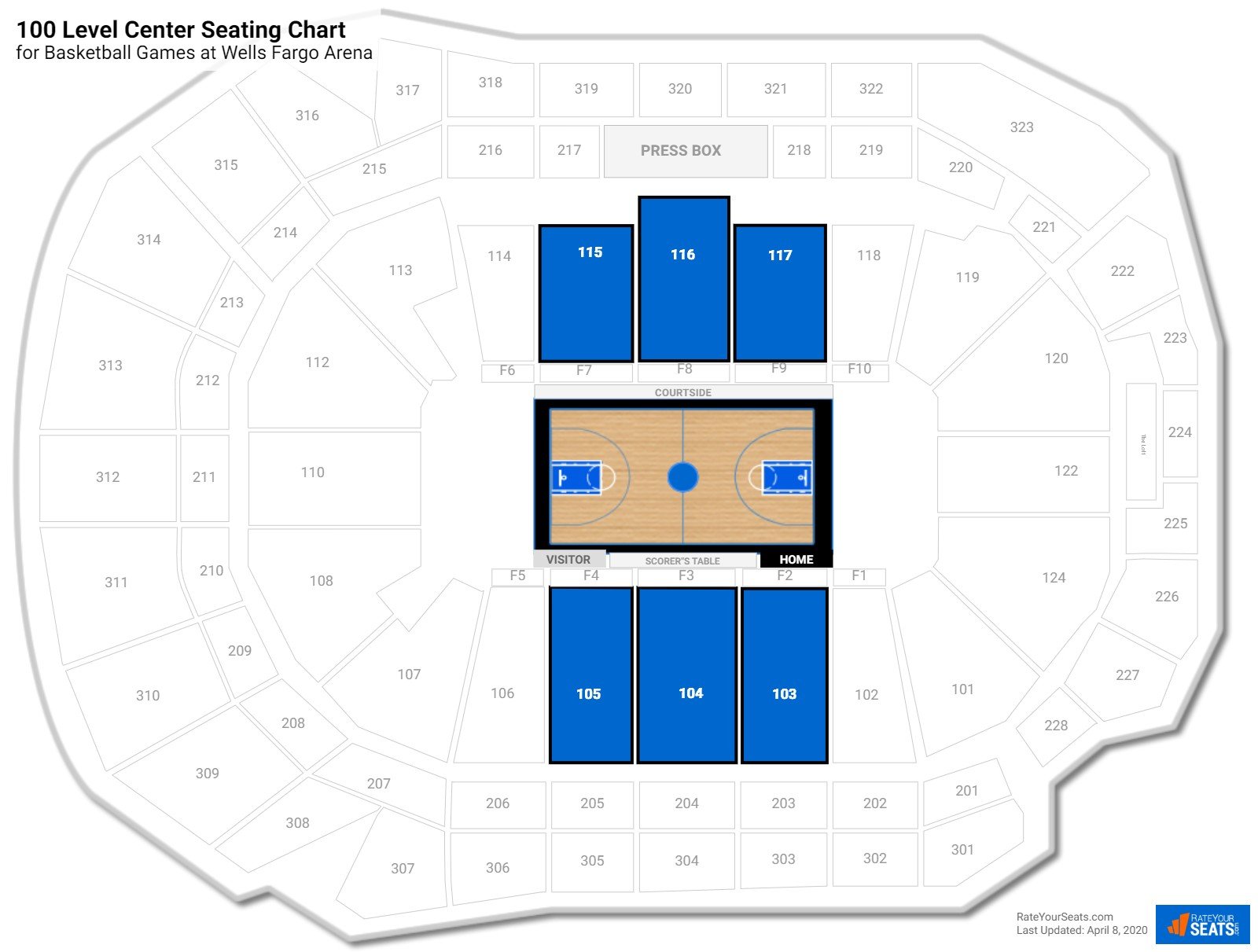The image depicts a detailed seating chart for basketball games at the Wells Fargo Arena. The diagram clearly outlines the various seating sections, starting with the "300" level at the top corners, commonly referred to as the "nosebleed" sections. These seats encompass the highest and farthest areas from the court, arranged in a circular pattern with labels such as "319" and "320," representing different sections within this tier.

Progressing inward, the "200" level seats are closer to the court than the "300" level, offering a better vantage point for spectators. As the chart shows, the "100" level seats are even nearer, providing excellent views of the game. These sections, closer to the action, are marked clearly in the middle tier.

At the arena floor level, the seats are prominently highlighted in blue boxes, distinct from the generic white and gray of the other sections. These prime seating areas seem to include only about six blue boxes, emphasizing their exclusivity and proximity to the court.

In the very center of the image, an icon illustrates the basketball court itself, complete with the typical markings and lines seen in professional NBA games, suggesting this chart is tailored specifically for NBA events. The layout includes views of both team benches and the key details relevant to the game.

Finally, towards the outer edges of the diagram, there is a small blue box containing an advertisement related to the arena seating, with a date listed as April 2020. This could indicate an event or promotion relevant to that specific period.